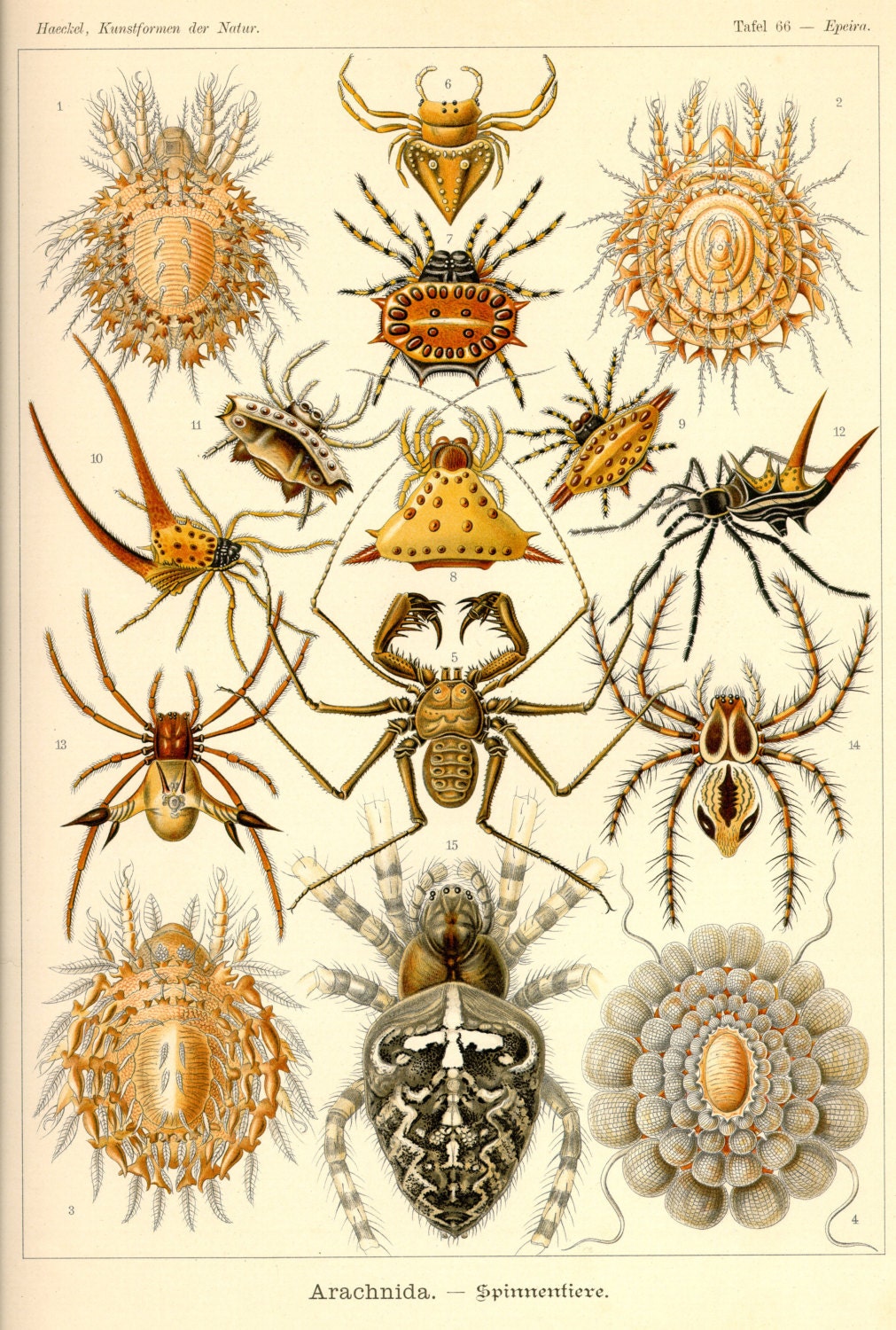The image depicts an old-fashioned, ornately illustrated diagram on an antique beige background, presenting various spiders and arachnids. In total, there are around 14-15 of these creatures, arranged in rows and columns, with numbering but no specific labels for identification. The arachnids are rendered in subdued colors, including tans, grays, browns, golds, and rusty reds, giving the diagram a muted yet detailed aesthetic.

At the very bottom of the page, in small black text, it reads "Arachnida-Spimeniter" (or a similar variant, the exact wording unclear), indicating the classification of the depicted spiders. The diagram is bordered by a thin black line, adding to its vintage presentation.

Unique features of the arachnids are detailed meticulously: from spiders with light gray and white striped legs to those with brown and mini gray legs. A particularly noticeable figure is a spider-like creature with a black body and red horns at its back end. Some of the illustrations include elaborate geometric designs, like shells with concentric rings leading to a central point, possibly a gold egg-like object.

Text at the very top of the page is partially legible and appears to be in another language, with phrases such as "Table 6-6" and possibly "Epsint." Despite the historical and somewhat decorative depictions of the arachnids, the intricate details suggest a blend of scientific and artistic endeavors typical of old natural history books.